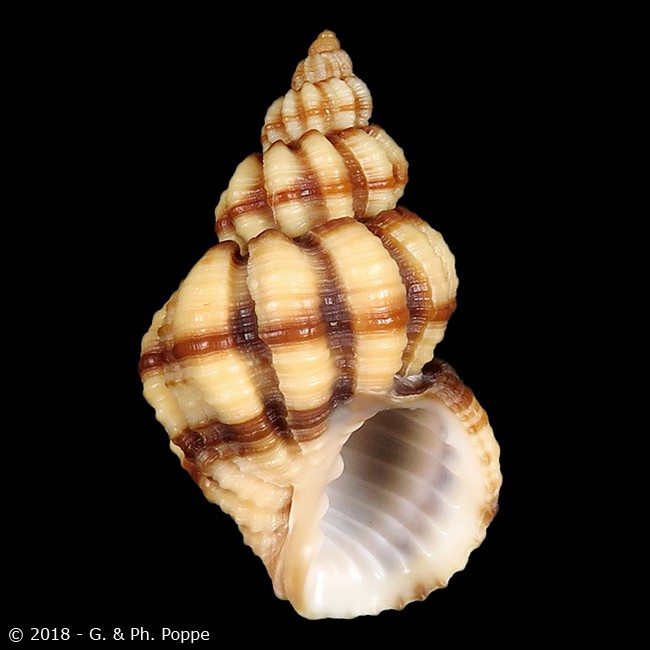This is a vertical rectangular image showcasing a detailed photograph of a seashell on a stark black background. The shell, centered in the image, is a yellowish-beige color featuring multiple rows of intricate scallops, with each row highlighted by a distinct brown stripe running through the center. The opening of the shell faces the lower right corner, revealing a white interior rimmed with hints of brown. The image exudes a dramatic and professional aura, potentially for a scientific or artistic context. In the lower left corner, the copyright text "2018 G.PH. Poppe" is clearly visible, emphasizing the photograph's meticulous curation and presentation.